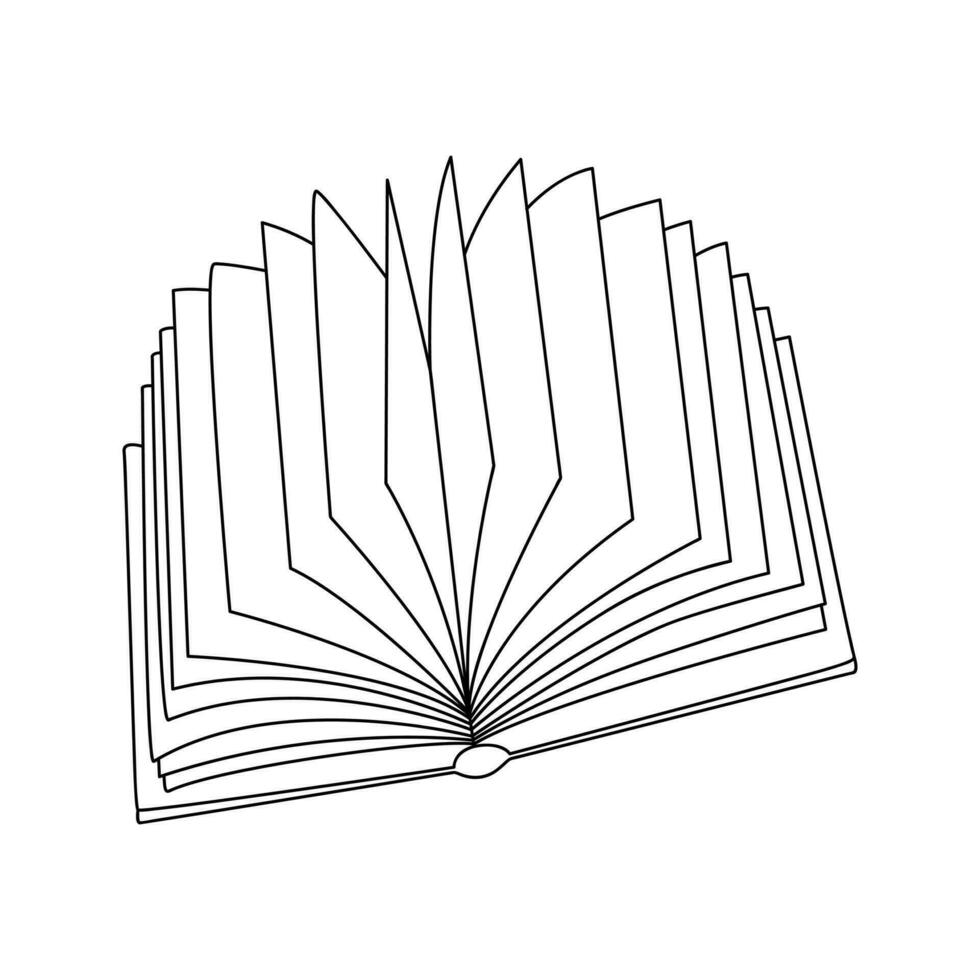This image features a meticulously drawn, symmetrical black line sketch of an open hardback book on a stark white background. The book, devoid of any decoration or color, reveals around 20 blank pages fanning out from the center, creating a geometric and orderly appearance. The pages, while appearing to flutter, remain unreadable due to their blankness. The entire scene is rendered in black and white, with no text, images, or embellishments, emphasizing the book's minimalist and angular design. The book is slightly tilted, around 15 degrees from the horizontal, adding a subtle dynamic to the otherwise serene and empty composition.